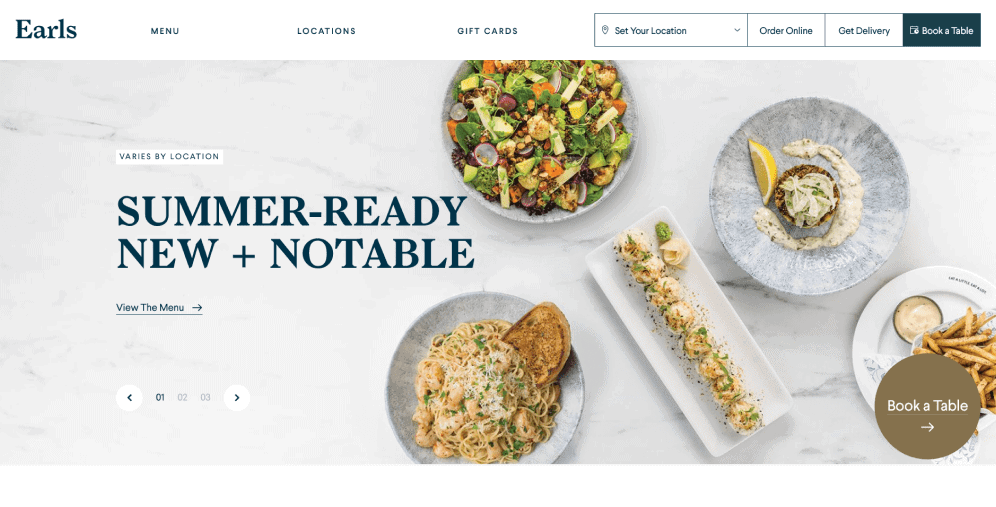The top left corner of the image features the title "Earl's" in a navy blue font, with a capitalized "E." Beneath this, in smaller, all-capitalized blue letters, it says "MENU." Adding to the navigation options, there are sizable spaces separating "LOCATIONS" and "GIFT CARDS." 

Towards the right, a rectangular box outlined in navy blue includes a map pin icon on the left, indicating the option to "Set Your Location" through a dropdown menu. Neighboring boxes include "Order Online," "Get Delivery," and "Book a Table," each with a navy blue background and white text.

Below this navigation section, a banner displays an elegantly set marble table adorned with an array of dishes. At the top, there's an avocado salad followed by a pasta shrimp dish on the left, complete with a piece of bread in the center. Adjacent to the pasta dish, a plate of sushi rests on a pristine white plate, and to the right, a decadent dessert is presented. Additionally, a serving of French fries accompanied by a dipping sauce is visible beneath these dishes.

To the left of the banner, a small white banner in navy blue letters reads "VARIES BY LOCATION" in small capitalized letters. Below, in larger, bolder navy blue capital letters, a seasonal promotion reads "SUMMER DASH READY NEW + NOTABLE." An interactive "View The Menu" option is underlined, with an arrow pointing to the right.

At the bottom of the banner, navigational controls are indicated by white circles on the left and right, allowing users to move between pages. Page indicators labeled 01, 02, and 03 denote the current page, with "01" highlighted in navy blue to signify its selection.